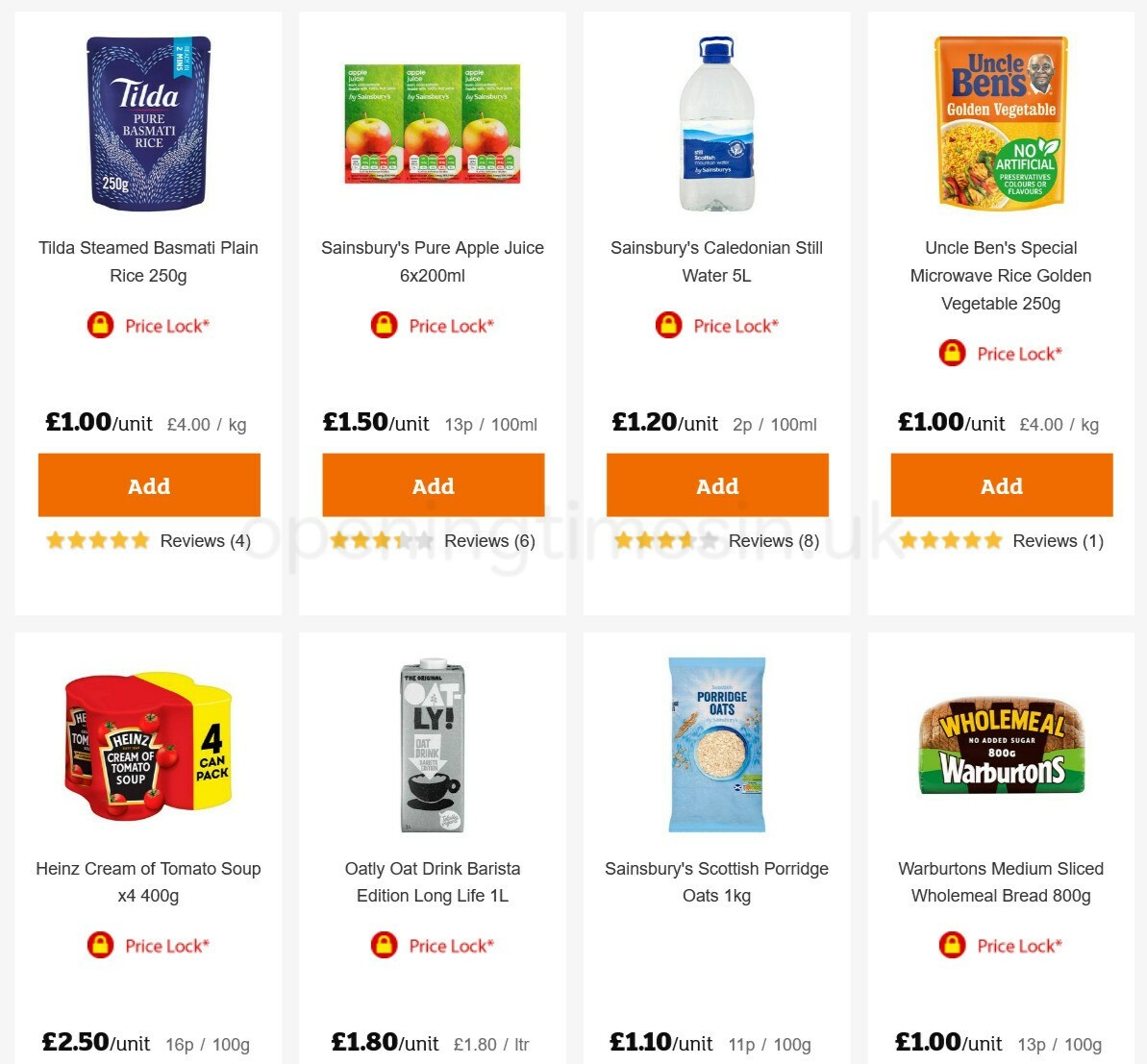Here is a cleaned-up and detailed caption for the given image:

---

The screenshot displays a well-organized web page featuring a variety of food items available for purchase. Each product is shown with clear and attractive images, set against a white background. The items listed include:

1. **Tilda Steamed Basmati Plain Rice** - Priced at £1.00.
2. **Pure Apple Juice** - Priced at £1.50.
3. **Sainsbury's Caledonian Still Water** - Priced at £1.20.
4. **Uncle Ben's Special Microwave Rice, Golden Vegetable, 250 grams** - Priced at $1.00.
5. **Heinz Cream of Tomato Soup, a 4-pack** - Priced at £2.50.
6. **Oatly Oak Drink Barista Edition Long Life, 1 Liter** - Priced at £1.80.
7. **Sainsbury's Scottish Porridge Oats** - Priced at £1.10 per unit.
8. **Warburton's Medium Sliced Wholemeal Bread, 800 grams** - Priced at £1.00 per unit.

Each item has an easily identifiable "Add to Cart" button, highlighted in orange. Review ratings are visible for some products, with scores ranging from 4 to 8, although the reviews for the last four items are partially cut off in the screenshot. Overall, the page is visually appealing and user-friendly, facilitating an enjoyable and straightforward shopping experience.